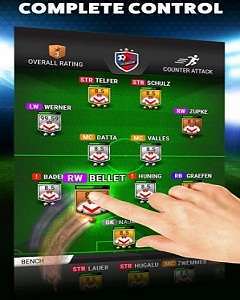This is an advertisement for a fantasy sports game, potentially featuring soccer or NFL football. The central focus is a top-down, simplistic view of a sports field. On this field, player icons for two teams are displayed, with one team's icons positioned at the top and the other team's icons at the bottom. Each player icon is labeled with a name. In the lower-right corner of the image, a light-skinned human hand is shown pointing and touching one of the player icons on the screen, indicating interaction with the game. At the very top of the image, in large white block letters, the words "Complete Control" are prominently displayed, emphasizing the game's user-friendly and interactive nature.